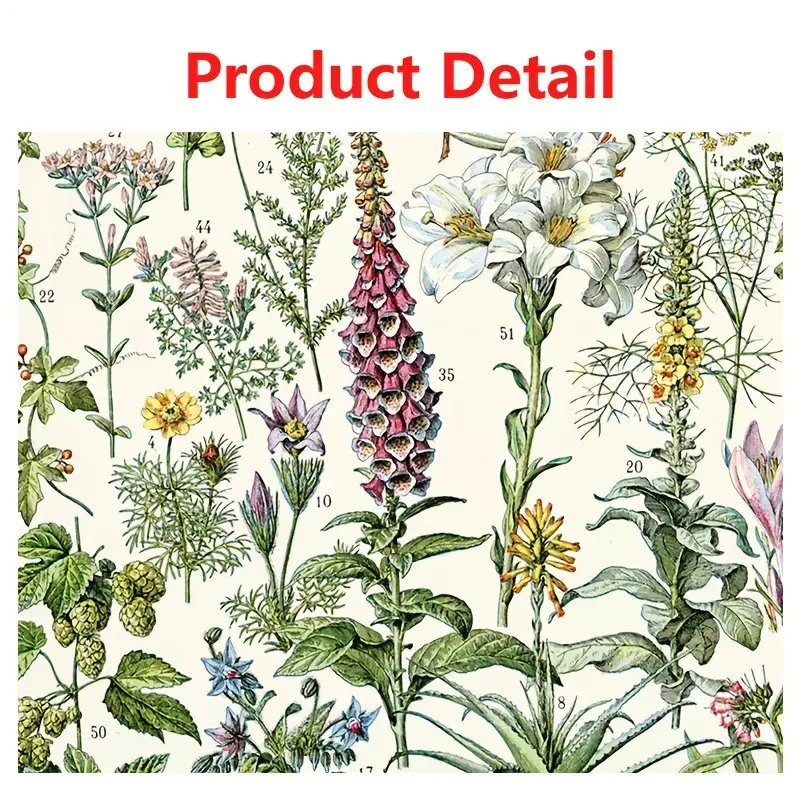The image features a rectangular illustration on a cream background showing detailed, color drawings of various flowering plants, each meticulously numbered in black for easy identification. The numbers 4, 8, 20, 35, 50, and 51 are discernible in the image. At the top of the image, the words "Product Detail" are prominently displayed in red font against the white background. The array of plants includes a tall stem of purplish-pink foxgloves labeled 35 at the center, surrounded by white lilies labeled 51, and a striking spike of yellow snapdragons labeled 20. A plant with clover-like clusters resembling hops, marked as number 50, and another plant with fiery red poker-like blooms labeled 8 add diversity to the collection. Smaller, pink lily-like flowers and a possible gerbera daisy, labeled 4, contribute to the rich array of botanical illustrations. These detailed plant drawings, resembling clip art, suggest the image may represent a product bundle available for design purposes, perhaps on platforms like Etsy.